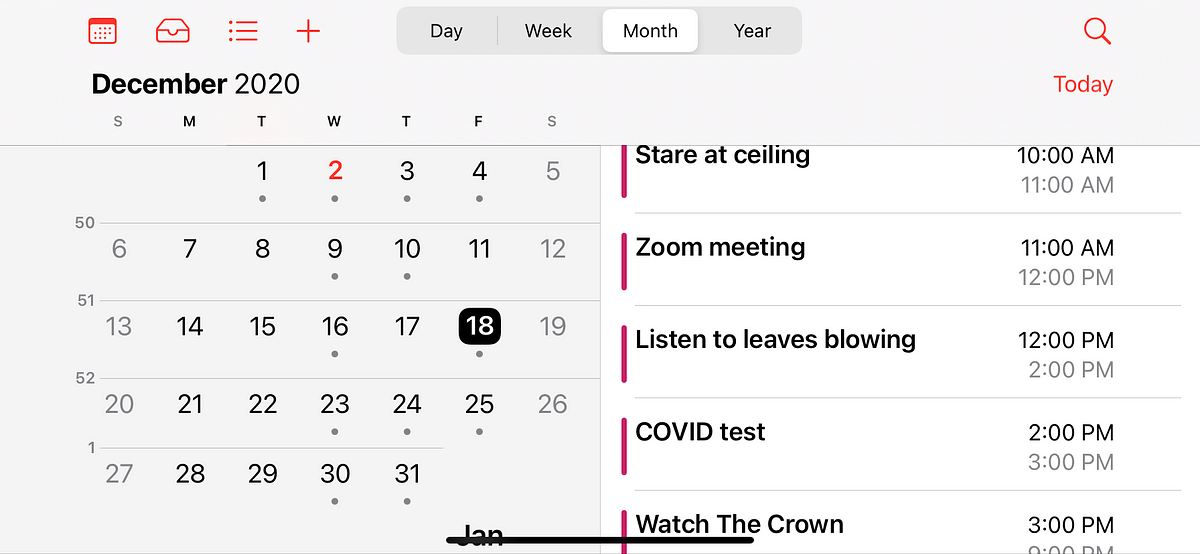This image is a screenshot of a digital calendar, which could be from either a laptop or a mobile device, as there are no clear indications of which it is. The calendar is set to December 2020. Specifically, December 18th, 2020, is selected. To the right of the calendar, a detailed schedule for December 18th is displayed. The scheduled items are as follows: 

- At 10:00 AM, there is an activity titled "Stare at the Ceiling."
- At 11:00 AM, there is a "Zoom Meeting."
- At 12:00 PM, the schedule lists "Listen to Leaves Blowing."
- At 2:00 PM, there is an appointment for a "Covid Test."
- Finally, at 3:00 PM, the schedule includes "Watch The Crown." 

This thorough schedule gives an insight into a mix of mundane, digital, and necessary activities planned for that specific day.